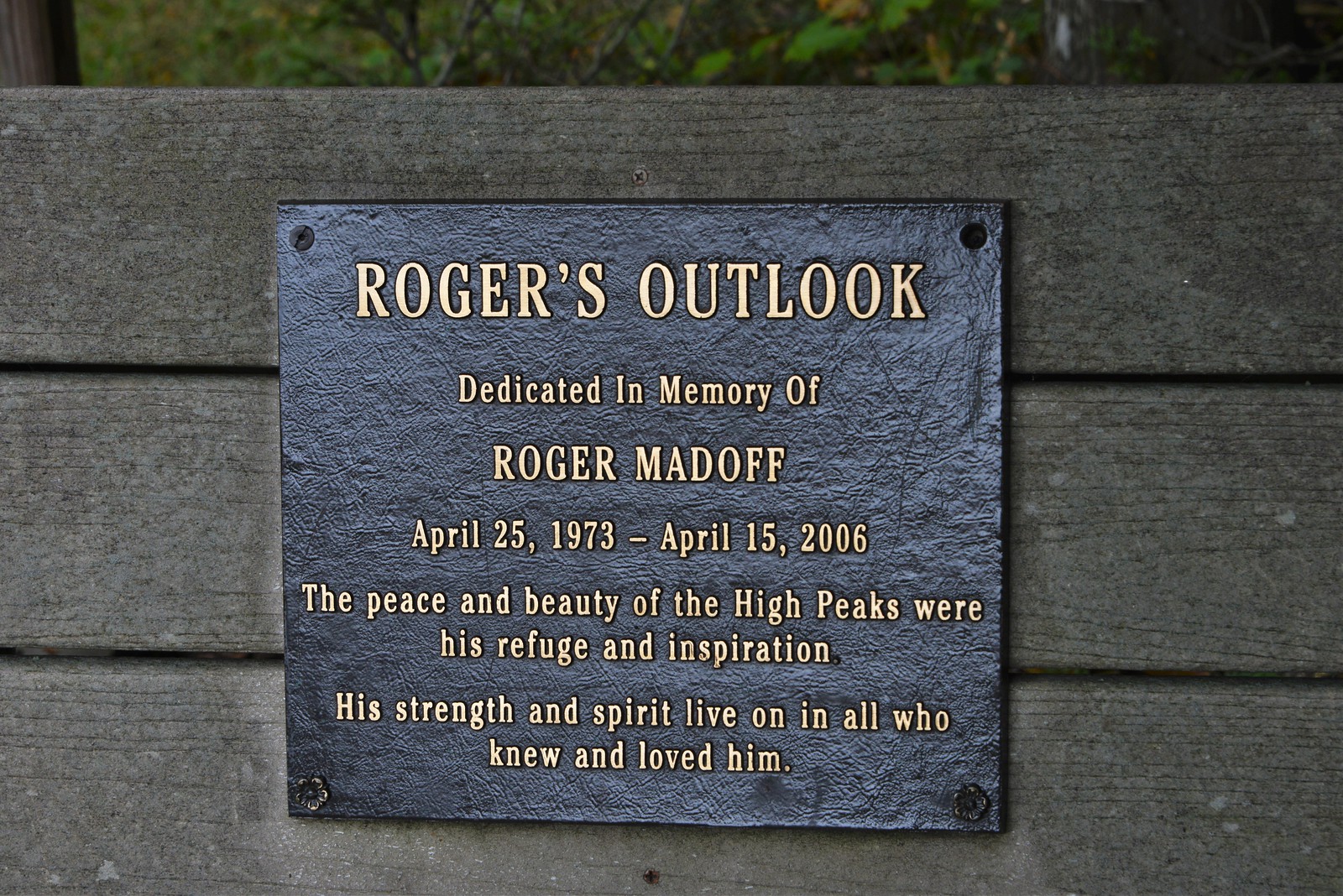This image captures a close-up of a memorial plaque mounted on dark gray wooden slats, with three boards visible. The plaque is black with golden lettering and is secured by screws at each corner. The text on the plaque reads: "Roger's Outlook, dedicated in memory of Roger Madoff, April 25, 1973 - April 15, 2006. The peace and beauty of the high peaks were his refuge and inspiration. His strength and spirit live on in all who knew and loved him." The background includes some green foliage, possibly part of a tree or tall grass, providing a serene natural setting that complements the memorial. The overall impression suggests that this spot, possibly connected to a bench, is intended for reflection and enjoying the surrounding beauty.